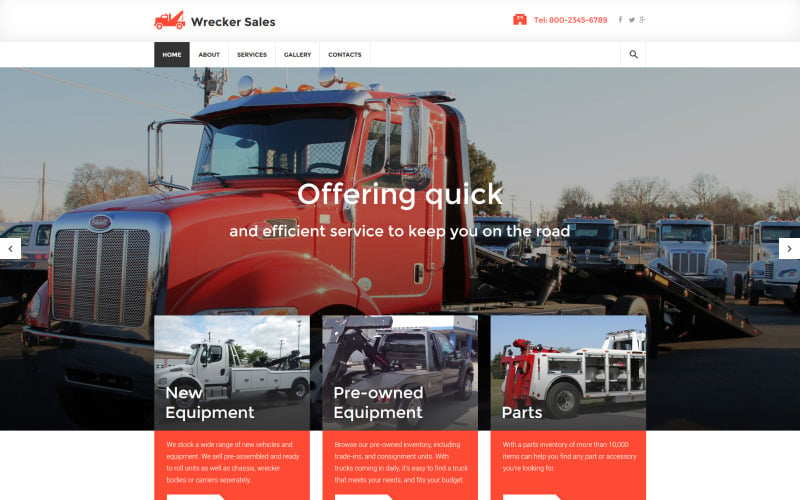The image depicts the homepage of the Wreckers Sales website. The top banner prominently features an orange-toned image of a pickup truck, accompanied by the site name "Wreckers Sales" in bold black font. Adjacent to this, on the right, is the telephone number 800-2345-6789. Social media icons for Facebook and Twitter are also visible, although the third icon is not clearly identifiable.

Below the banner, there is a navigation bar with tabs labeled Home, About, Services, Gallery, and Contacts, along with a search key on the far right. The Home tab is highlighted in white font against a black background, while the other tabs are displayed in black font.

Central to the page is a large image showcasing an orange flatbed tow truck. Superimposed on this image is the slogan in white font: "Offering Quick and Efficient Service to Keep You on the Road."   

Beneath this main image, a featured section displays three types of tow trucks:

1. "New Equipment" - Illustrated by a white pickup truck, with descriptive text on an orange background.
2. "Pre-Owned Equipment" - Depicted by a gray pickup truck, also with accompanying text on an orange background.
3. "Parts" - Shown with a white pickup truck featuring a red bed, with relevant text on an orange background.

The backdrop of the main photo reveals a serene scene of green trees and a collection of white and gray pickup trucks, set against a slightly overcast, gray sky.